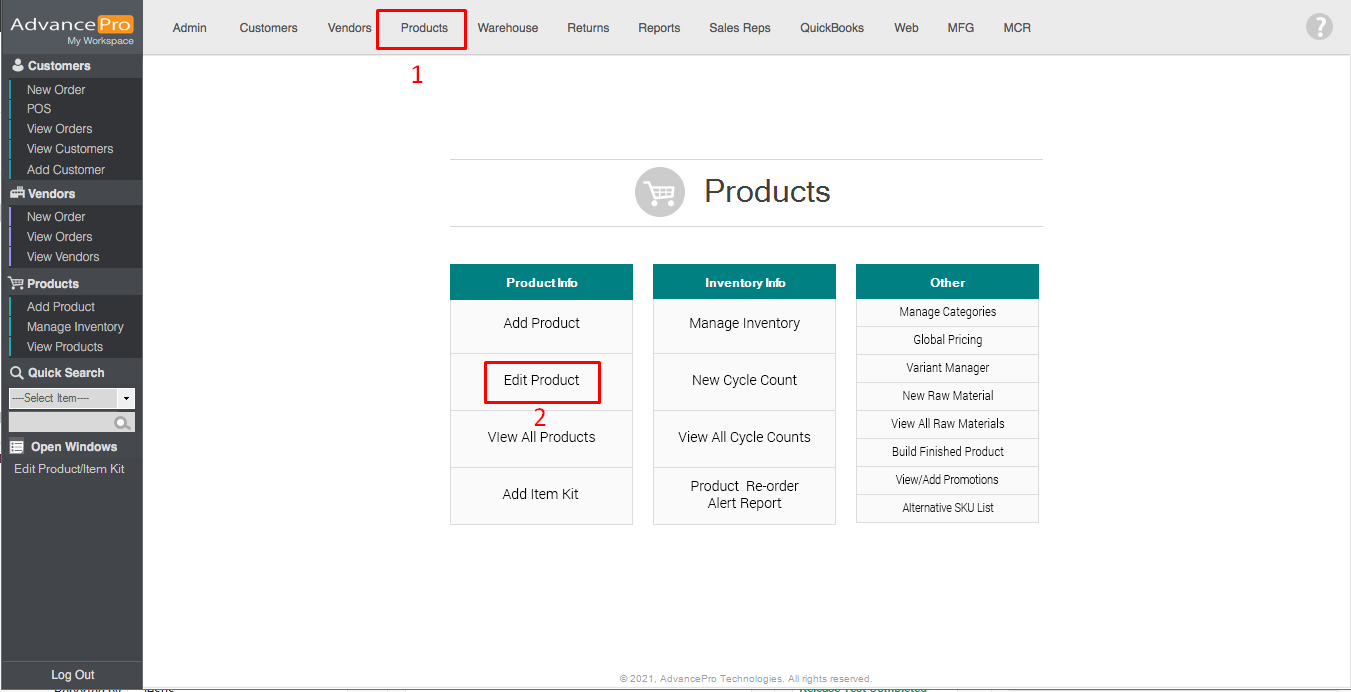The image displays a software interface with a detailed navigation menu and various options for managing products, customers, vendors, and inventory. The interface has a monochromatic theme consisting mainly of shades of gray, with some sections highlighted in purple and teal. 

At the top of the interface, the background is gray with the darker gray section towards the left-hand side. The title "Advanced" is prominently displayed in white text within this darker area. On the right-hand side, there is a white box labeled "Pro," which likely indicates the version of the software.

Below the header, the interface prominently displays several main menu options:
- **My Workplace**: This section includes sub-options such as "Customers," "New Order," "POS View," "Orders," "View Customers," "Add Customers," and "Vendors."
- **Orders**: This section is highlighted with a purple left-hand side and includes options like "New Order," "View Orders," and "View Vendor."
- **Products**: This section has a teal-colored left-hand side and offers options like "Add Product," "Manage Inventory," and "View Products."

A quick search feature is available, marked by a white magnifying glass icon, with an adjacent gray search box labeled "Search Items." Below this, another gray box with a magnifying glass icon is labeled "Open Windows."

The bottom of the interface features a white horizontal line with the option to "Logout."

Below these, a gray section lists additional options including "Admin," "Customers," "Vendors," and "Products." This section has a red square box around it with further categories like "Warehouse," "Returns," "Reports," "Sales Reps," "QuickBooks," "Web," "MFG," "MCR," "Product Info," "Inventory Info," and "Other." The "Other" section displays sub-options like:
- **Add Product**: In black text with a red box and the number "2" underneath.
- **Edit Product**: Also in black text with a red box.
- **View All Products**
- **Add Item** and **Add Item Kit**
- **Manage Inventory**, which includes options like "New Cycle Count," "View All Cycle Counts," and "Product Reorder Alert Report."
- **Manage Categories**, "Global Pricing," "Variant Manager"
- **New World Materials**, "View All World Materials," "Build Finished Product," "Review/Add Promotions," and "Return SKU List."

This in-depth interface is tailored for comprehensive management of business processes, ensuring users have access to a wide range of functionalities from adding new products to managing inventory and customer information. The visual design features color-coding and boxed elements to distinguish different sections and functions, enhancing user navigation and experience.